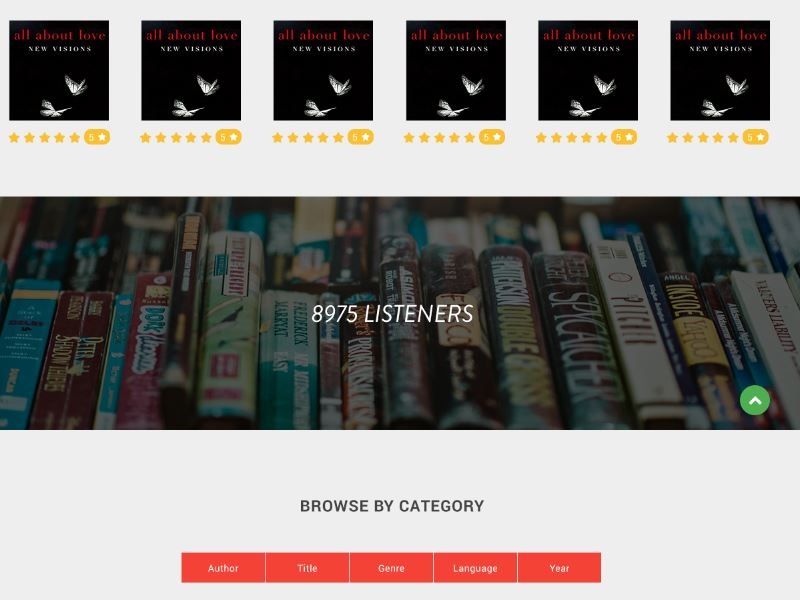The image depicts a website layout featuring what appears to be the cover of an album, repeated six times horizontally across the screen. Each album cover is set against a black background and showcases two butterfly-like images, one seemingly in flight and the other about to land. These elements form the centerpiece of the display.

At the top of each album cover, a title is prominently displayed in red lettering, presumably the name of the album. In front of each cover, a five-star rating is visibly shown, indicating high user satisfaction. 

Beneath the album covers, there is a vertical section featuring the spines of various books, each adorned in vibrant colors like pink, green, and blue, with different titles displayed. This section includes text stating "8,975 listeners" in white, suggesting user engagement metrics.

In the lower right-hand corner, a green arrow icon is visible, possibly indicating a navigational or interactive feature. Below this area, a gray box houses the text "Browse by category," followed by red rectangular boxes listing categories such as "Author," "Title," "Genre," "Language," and "Year" at the very bottom of the image.